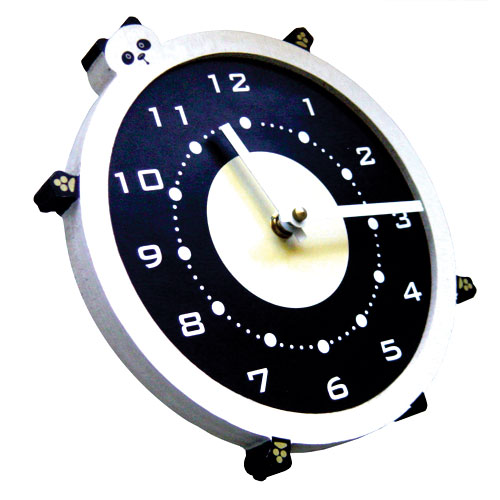This charming alarm clock features an endearing panda design, where the main timepiece—complete with Arabic numerals—is encased within a whimsical panda figure. The hour and minute hands are positioned between the 11 and 12 and pointing at 3, respectively. The outer rim of the clock is fashioned like a plush, round panda body, with a small, adorable panda face peeking out above the 11 and 12 positions. Tiny panda arms extend from its body, adding to its playful and cuddly aesthetic. At the bottom of the clock is a supportive piece designed for stability, allowing it to lean comfortably on any surface. This delightful timepiece makes for a perfect and cute gift, sure to bring a smile to anyone's face.